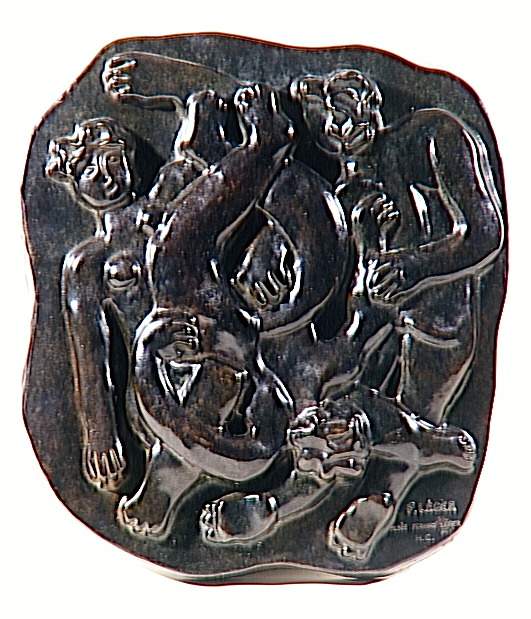This image depicts a highly intricate and shiny metallic artwork, possibly crafted from a dark gray or silverish metal with hints of brown. The piece, which resembles a carved metal plaque or coin, features detailed carvings of human figures in deep relief. At the center, there is a dramatic scene of a man entangled in a fierce wrestling match with a creature that appears to be a hybrid of a dragon or lion, possessing a human-like form with distinctive paws. A woman is positioned to the left of the scene, adding to the complexity of the composition. The figures, with their thick limbs and bodies intertwined in a snake-like pattern, are set against a backdrop of intricate metalwork. This central tableau captures a moment of intense struggle and movement, highlighting the artist's skill in depicting dynamic and intertwined forms.